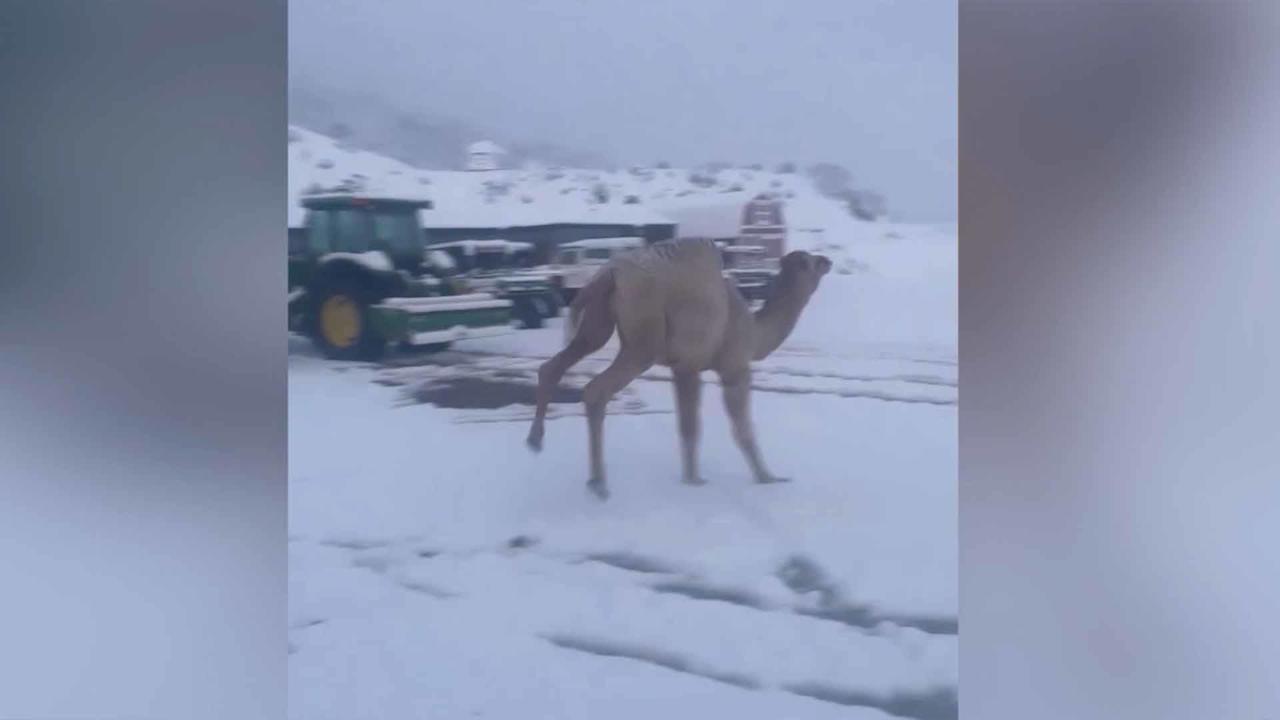This image depicts a brown, one-humped camel standing outside in a snowy terrain. The setting appears to be somewhat blurry, with tracks from vehicles visible in the snow-covered foreground. The background is dominated by a gray, somewhat ominous sky that hints at an ongoing or impending snowfall. A green tractor with black tires and some snow on it is prominently visible, along with a variety of other vehicles, including a truck and a jeep. To the right of the camel, there's a small puddle of brown water. Further in the background, there's a gray barn with snow on its roof, and hills blanketed in snow with sparse shrubs and bushes protruding through. The overall scene conveys a stark, wintry landscape with the unusual sight of a camel navigating through the snow.